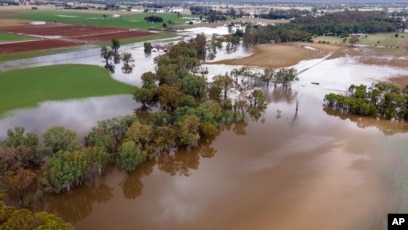The image depicts an aerial view of a flooded farmland landscape. Dominating the right side and part of the background is a large, murky brown lake resembling overrun swampy waters. On the left side of this lake, a line of partially submerged trees stretches towards the center of the image, forming a zigzag pattern that shifts left and right as it moves back. To the left, across these trees, there is a small patch of green land, behind which lies a smaller, separate lake nestled between additional parcels of land. In the upper left corner, fields of a brown hue can be seen, while adjacent areas show patches of greenery, tree clumps, and lighter green grass. The red field mentioned adds complexity to the mid-ground, and small buildings are faintly visible on the distant horizon. Low-lying structures can be observed in the upper left-hand corner, suggesting a marshy, flood-prone environment, perhaps indicative of typical Midwestern topography. The lower right corner of the image contains a watermark with the initials "AP."